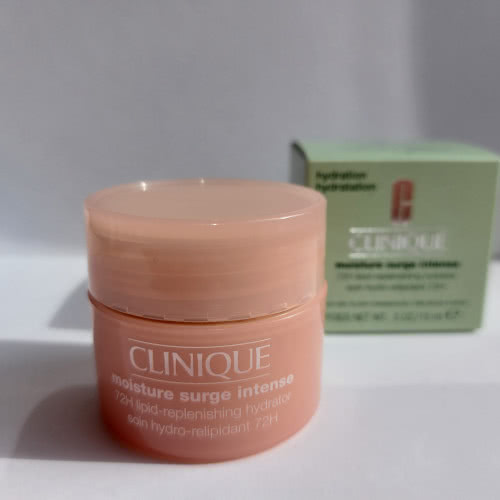In the image, a prominently displayed small pink bottle is showcased in the forefront. The bottle, which appears to be a glass jar with a plastic lid, contains a skin cream labeled in white font as "Clinique Moisture Surge Intense 72H Lipid Replenishing Hydrator" with additional details in a different language. The cream inside the bottle has a pink or salmon hue. Positioned behind and slightly to the right is an out-of-focus green box, also branded with the Clinique logo in silver font and some additional, undecipherable black lettering. The entire setup rests on a gray surface and is set against a gray background, which emphasizes the shadows cast to the left by the products. The scene seems to be a stock photo likely used for a Clinique advertisement.